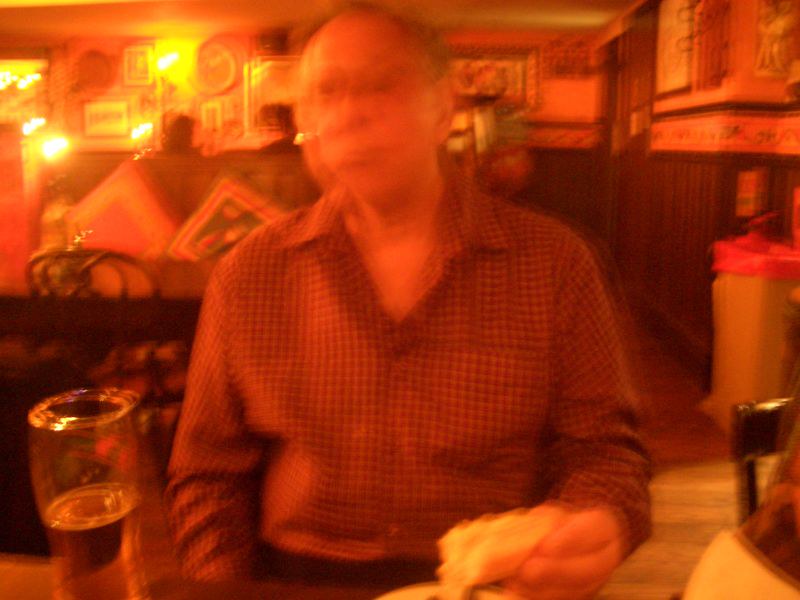In this softly-focused image of a cozy restaurant or bar, a man dressed in a red and black plaid shirt with small checks is seen enjoying a sandwich. He sits in a warmly lit seating area with a wooden floor and half-wooden walls up to a chair rail. The man holds a beer in a pilsner-style glass while savoring his sandwich. In the background, ambient amber lighting casts a pleasant glow over the space, complementing the decorative items adorning the distant walls. Another table and additional diners can be spotted faintly among the inviting interior, adding to the charming and lively atmosphere of the restaurant.